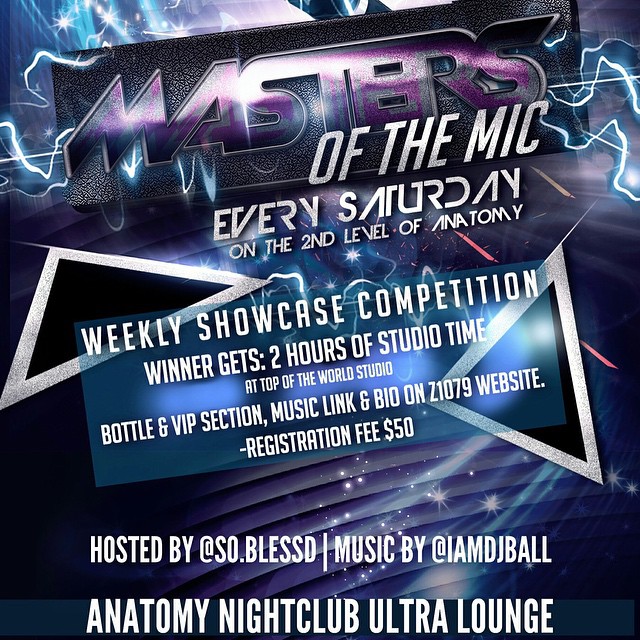This vibrant club flyer features an electrifying design with a black background accented by purple, blue, and white elements. The bottom portion showcases horizontal stripes in purple, while the top displays striking blue lightning bolts emerging from the sides of a central black, leather-like rectangular shape emblazoned with the word "MASTERS" in bold purple letters. Beneath this, in crisp white text, it announces "Masters of the Mic," an event occurring every Saturday on the second level of Anatomy Nightclub Ultra Lounge. 

The flyer highlights a weekly showcase competition where the winner is awarded two hours of studio time at Top of the World Studio along with a bottle and VIP section, with further details accessible via a music link and bio on the Z1079 website. Additionally, there is a registration fee of $50. The event is hosted by @so.blessed, with music provided by @IAMDJBALL.